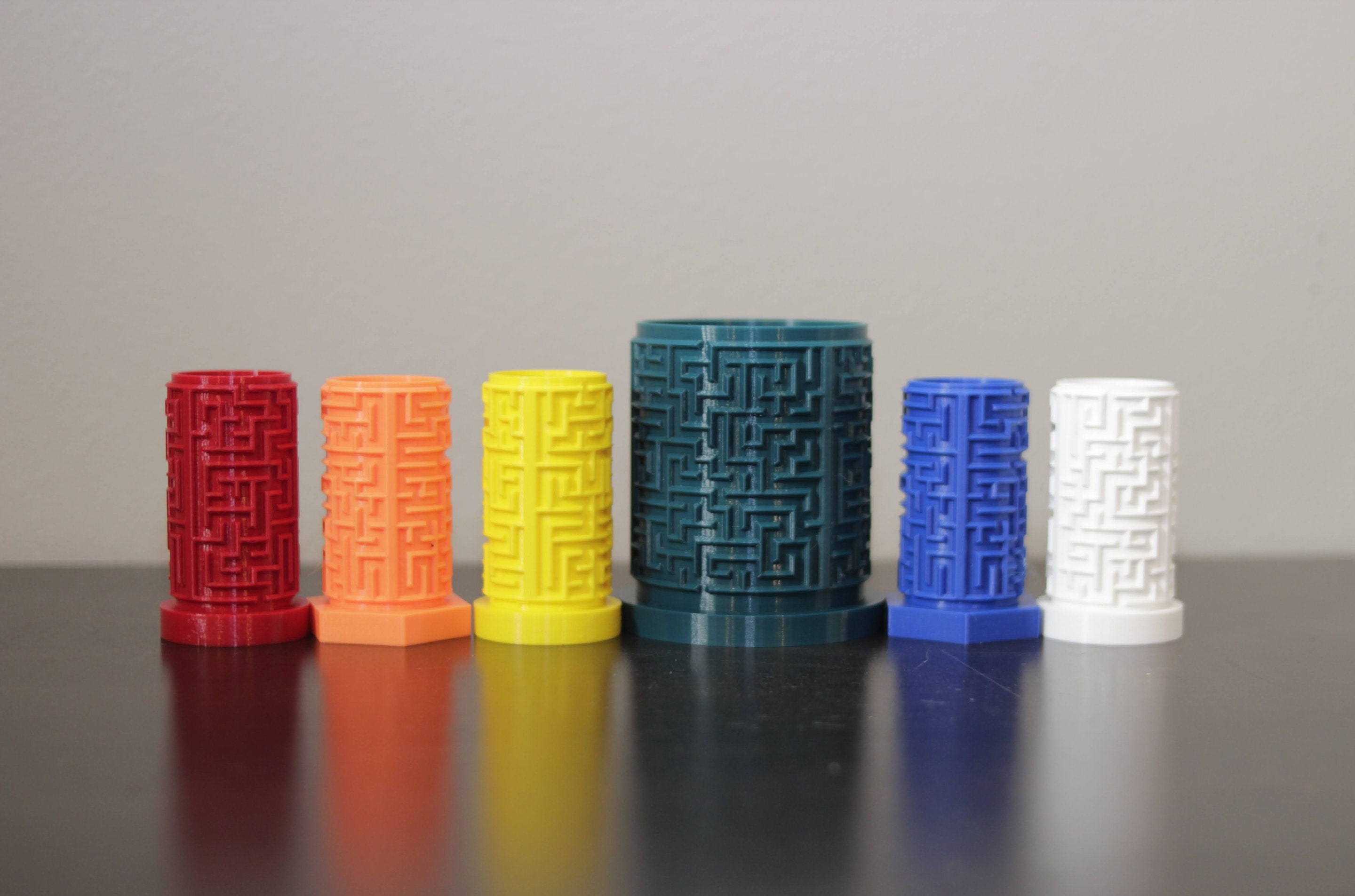The photograph features six 3D-printed cylindrical mazes, each in a distinct color and shape, displayed on a dark-colored, reflective table with a gray wall as the backdrop. From left to right, the mazes are detailed as follows: the first maze is red with a circular base and hollow top; the second is orange with a hexagonal base; the third is yellow with a circular base; the fourth and largest maze is a greenish-blue cylinder, notably taller and wider than the others; the fifth maze is blue with a hexagonal base; and the sixth maze is white with a circular base. Each maze is intricately carved, emphasizing their maze-like patterns. The dark table surface creates a mirrored reflection of the mazes, adding depth to the image.